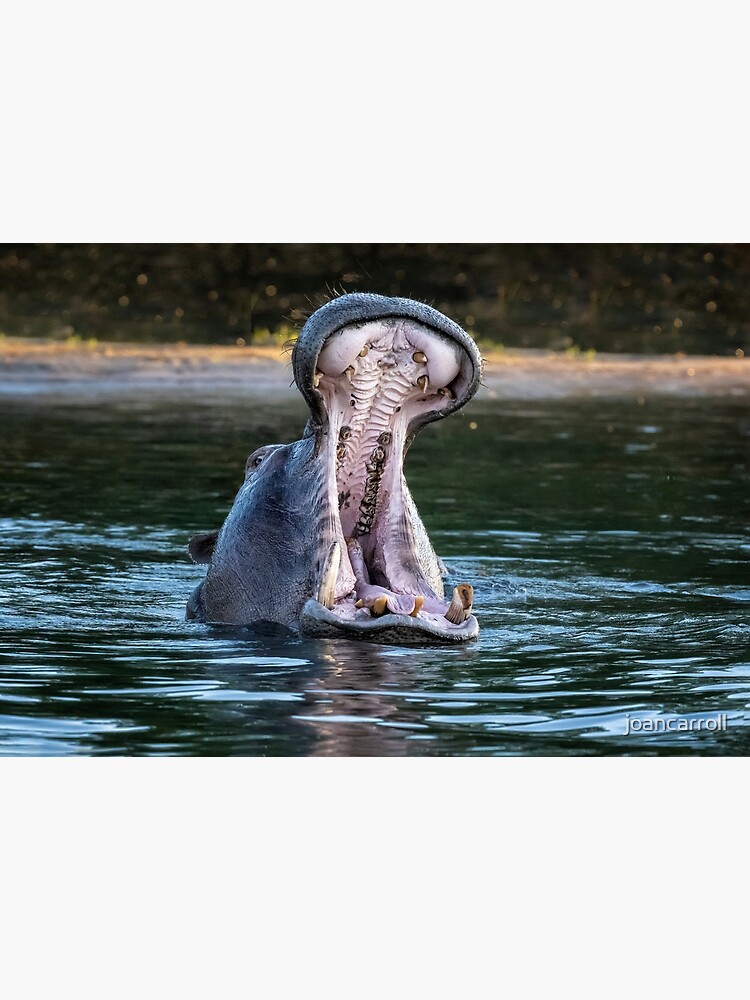The image captures a large hippopotamus in murky green water with its head tilted back, exposing its wide-open mouth. The close-up view allows a detailed look inside the hippo's expansive mouth, revealing several yellowish teeth that resemble tusks. You can also see the white roof of its mouth with crevices. Only the head is visible above the surface, showing one eye and one ear on the left side, enhanced by the soft ripples in the water around it. The serene water contrasts with the sandy bank and lush green plants in the background, indicating the hippo is in a lake or similar natural habitat. The bottom right corner of the image features the credit "Joan Carroll" in white text, lending credit to the photographer. The ambient light and reflections suggest it is daytime, creating an overall tranquil yet striking scene.